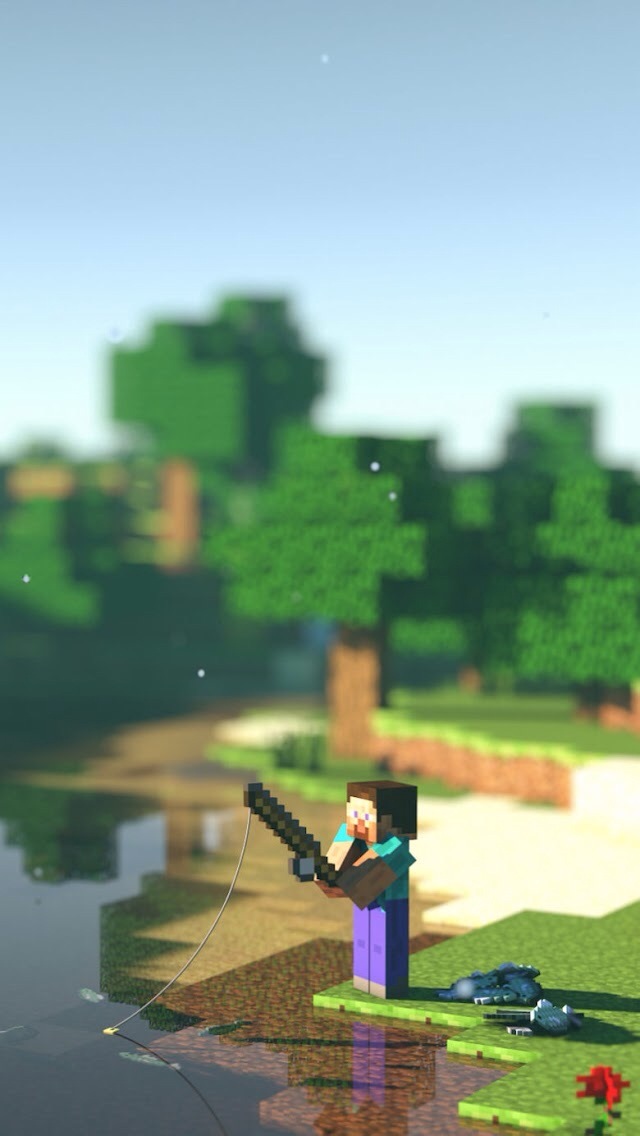An artistic screenshot from the game Minecraft shows a serene evening scene enhanced with a shader pack or RTX graphics, adding realistic lighting effects. The sky transitions from a deep dark blue at the top to a lighter blue and finally to a soft white near the horizon, suggesting the sun is setting. The blocky nature of Minecraft is preserved, with oak trees featuring lush green leaves and a mix of dirt and sand on the ground. A small red flower adds a splash of color to the otherwise earthy landscape. In the center stands a blocky character holding a pixelated fishing rod, showcasing a proud catch of several fish. Reflective water in the foreground mirrors the surrounding trees and sky, amplifying the tranquil beauty of the scene.